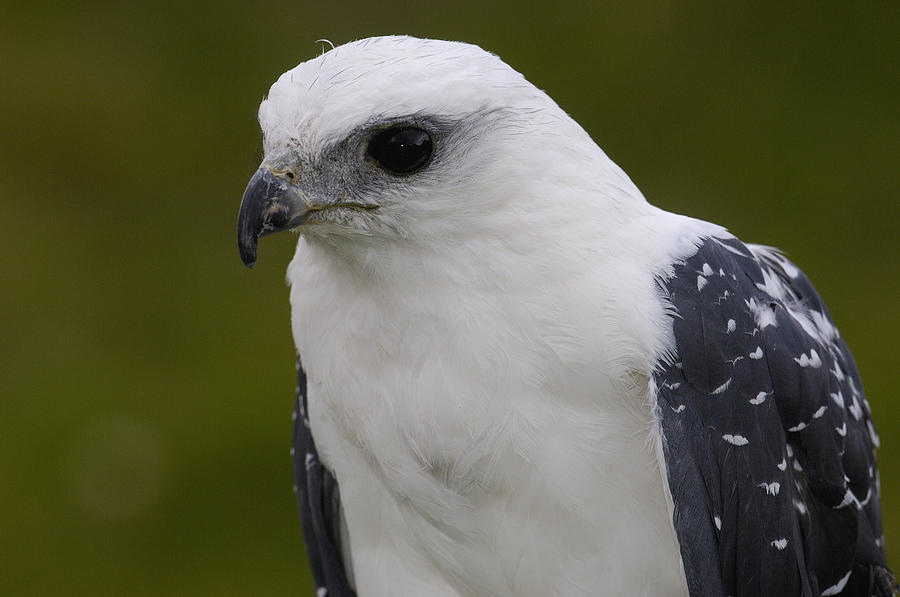In this high-resolution photograph, the central focus is a striking bird, possibly a hawk, set against a lush, blurry green backdrop that ranges from lime to hunter green. The image captures the bird from head to just over half of its body, with its beak and tail not visible. The bird’s head is slightly turned, displaying its left eye prominently at the front of the frame. Its eye is a dark, beady black, mirroring the color of its sharply curved beak. The bird's plumage is predominantly stark white, featuring short feathers on its body and longer wings adorned with black and gray tones and white specks near the tips. The wings are folded neatly against its sides, and the individual feathers can be discerned, underscoring the clarity and detail of the image. The overall composition highlights the bird's majestic appearance and the vivid yet blurred greens of its natural environment.